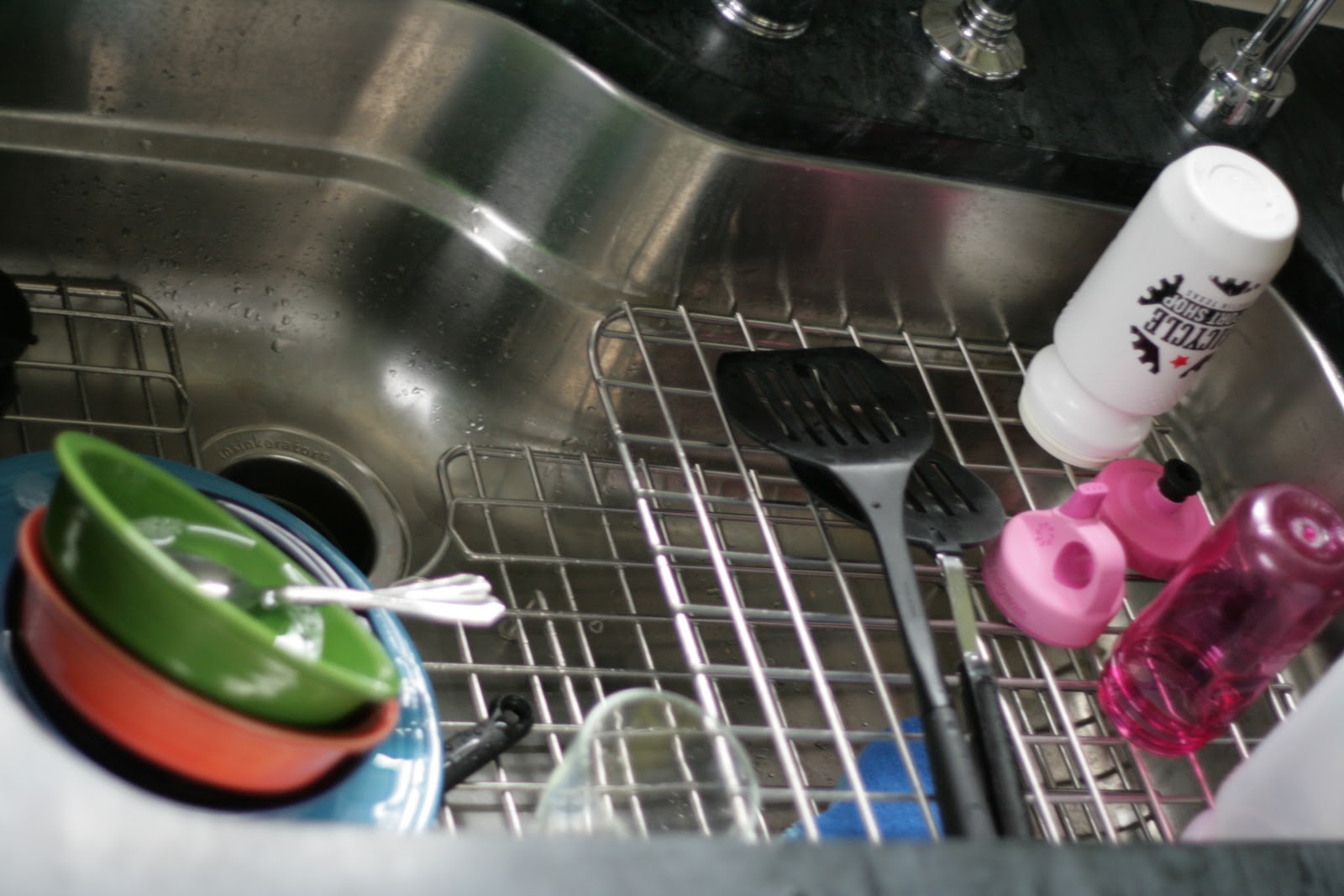The image showcases a kitchen sink, predominantly silver in color, situated within a black, possibly marble countertop. To the left side of the sink, a green bowl with two silver spoons lies adjacent to a red bowl resting inside a larger blue plate. The sink contains metal racks and, positioned to the right, two black spatulas. An upside-down white bottle with black lettering is also visible in this area, accompanied by two pink drinking lids—one with a black top and the other entirely pink—alongside an upside-down pink plastic bottle. Peeking at the base of the countertop are what appears to be silver taps. Beneath the racks, on the left side of the sink, there is a clear glass, and on the right side, a blue sponge sits on the silver sink surface.